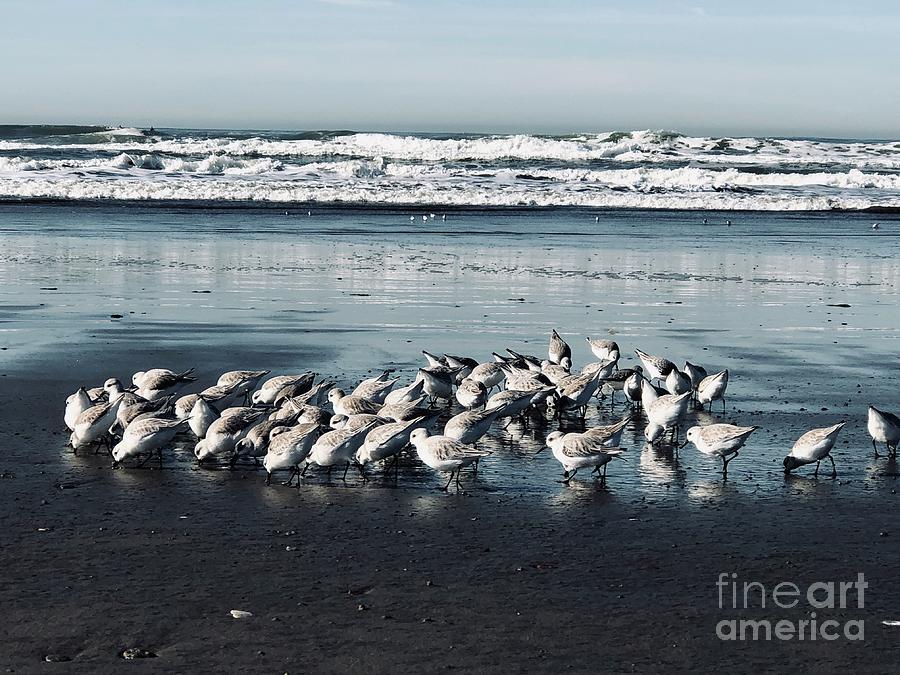This detailed photograph, with a watermark reading "Fine Art America" in the bottom right corner, showcases a dynamic scene at the ocean's edge. The foreground is filled with dark, wet sand, providing a striking contrast to the cluster of approximately 30-50 white seabirds with gray wings, long skinny dark legs, and slender dark beaks. These birds, resembling plovers or a similar shorebird species, are engaged in various activities. Many are seen burying their beaks into the sand in search of food, while others wander with their beaks up. In the middle ground, the sand transitions to the shoreline, where the tumultuous waters of the ocean crash against the shore under a sky adorned with thin, wispy gray clouds. In the distance, more seagulls can be spotted near the surf line. This photorealistic image could easily be mistaken for a piece of fine art, capturing the raw beauty and subtle complexity of nature.